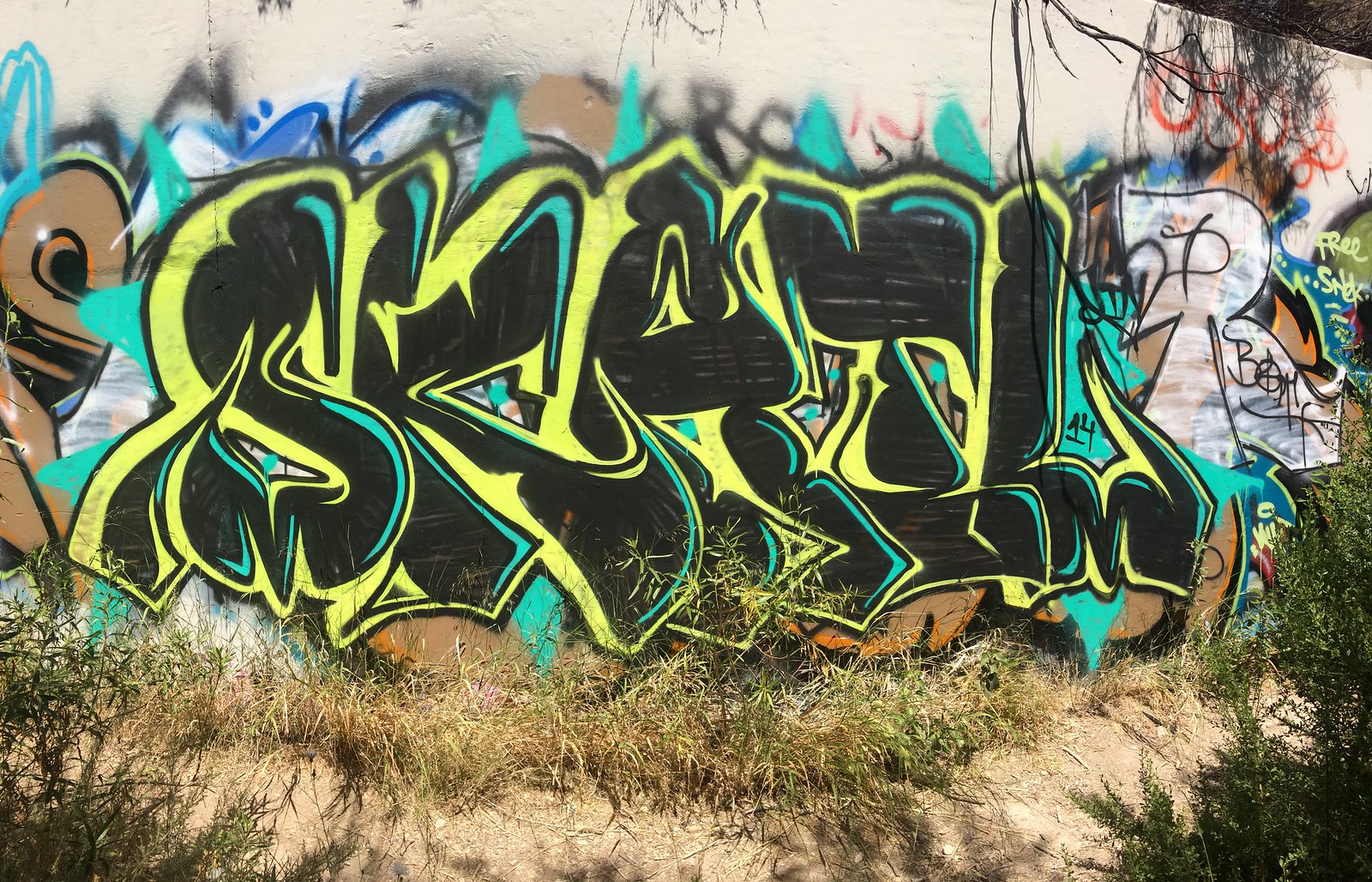The image captures a prominent piece of graffiti featuring the word "SKATL" in large, bold black bubble letters, accentuated with light blue highlights and outlined in a striking yellow border. This vivid artwork is displayed on a substantial white retaining wall, which appears to have painted over previous layers of graffiti. The older graffiti peeking through the new piece includes beige and blue elements, with some brown and black outlines, suggesting a similar lettering style. At the top corner of the wall, red graffiti is also visible. The scene is set in an outdoor environment with scraggly grass and patches of dirt in the foreground, along with a few branches hanging down from the top of the image. The overall setting includes a mix of urban decay and natural elements, against the backdrop of a slightly dirty and weathered wall.